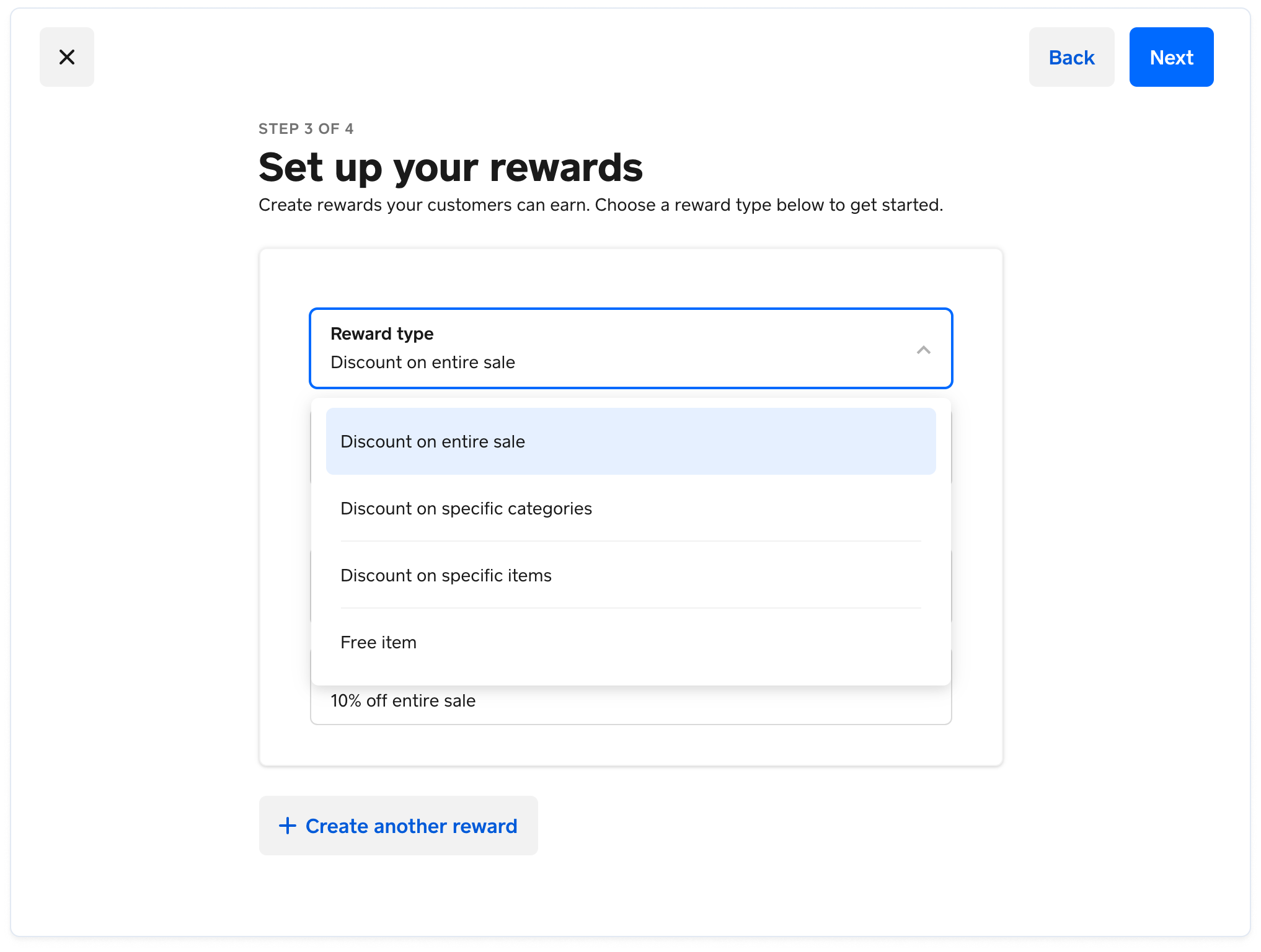A digital image showing Step 3 of 4 in setting up rewards for customers. The instructions are displayed in bold black font: "Create rewards your customers can earn. Choose a reward type below to get started." The first reward type, "Discount on entire sale," is highlighted in a blue rectangle, indicating that it has been selected. 

Beneath it, additional reward type options are listed, including "Discount on specific categories," "Discount on specific items," and "Discount on per-item option." An example reward of "10% off entire sale" is provided.

At the bottom of the image, a grey button with a blue plus sign invites users to "Create another reward." In the upper-left corner, an 'X' icon is visible for closing the screen. To the right, a grey "Back" button and a blue "Next" button are positioned in the lower-right corner to navigate through the setup process.